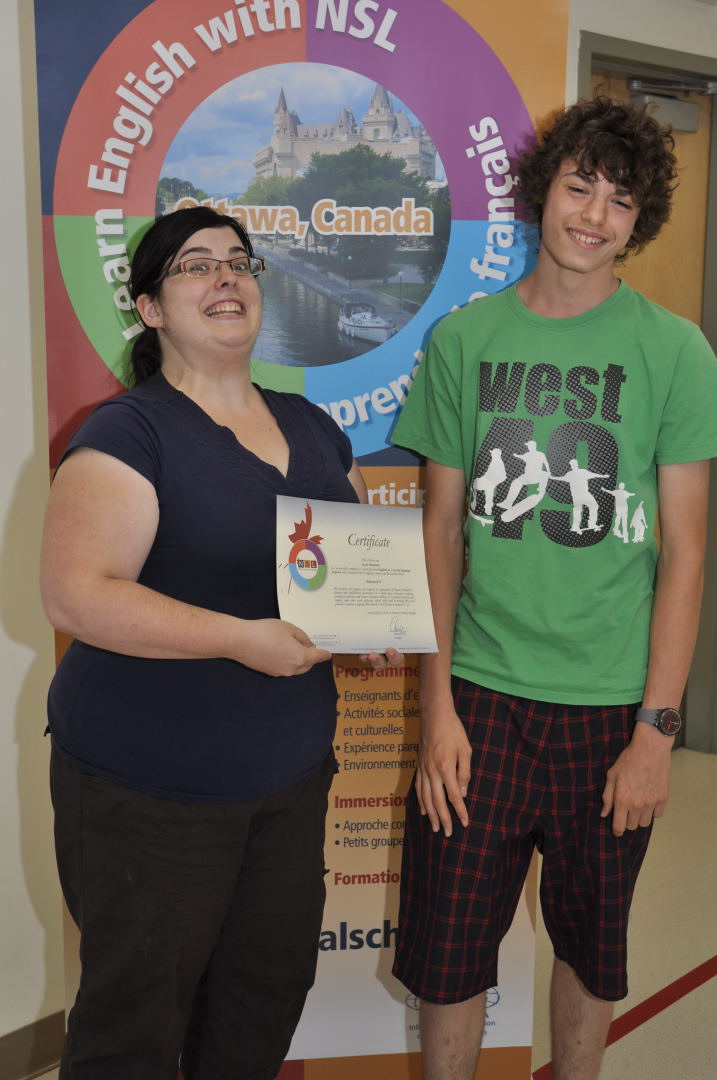In this photograph, a middle-aged woman and a young adult man stand in front of a banner, which is situated next to a wooden door on the right side of the image. The woman, who has black hair, wears glasses, and is smiling, stands on the left. She is dressed in a blue shirt and black pants, and she is holding a white certificate with both hands. The certificate features a circular design on the left side of its edge, divided into four colored quarters: top-left in orange, top-right in purple, bottom-left in blue, and bottom-right in green.

The young man on her right, with short curly hair, is wearing a green t-shirt with the word "West 49" in black font across his chest, accompanied by a white outline of someone skateboarding. He also sports a watch on his left wrist and black and red checkered shorts. The background shows a banner that reads "Ottawa Canada" in the center, with an image resembling a castle behind the text. The outer circle of the banner includes phrases like "France, English with NSL," among other writings. They appear to be standing in a school building characterized by white walls and an orange door.